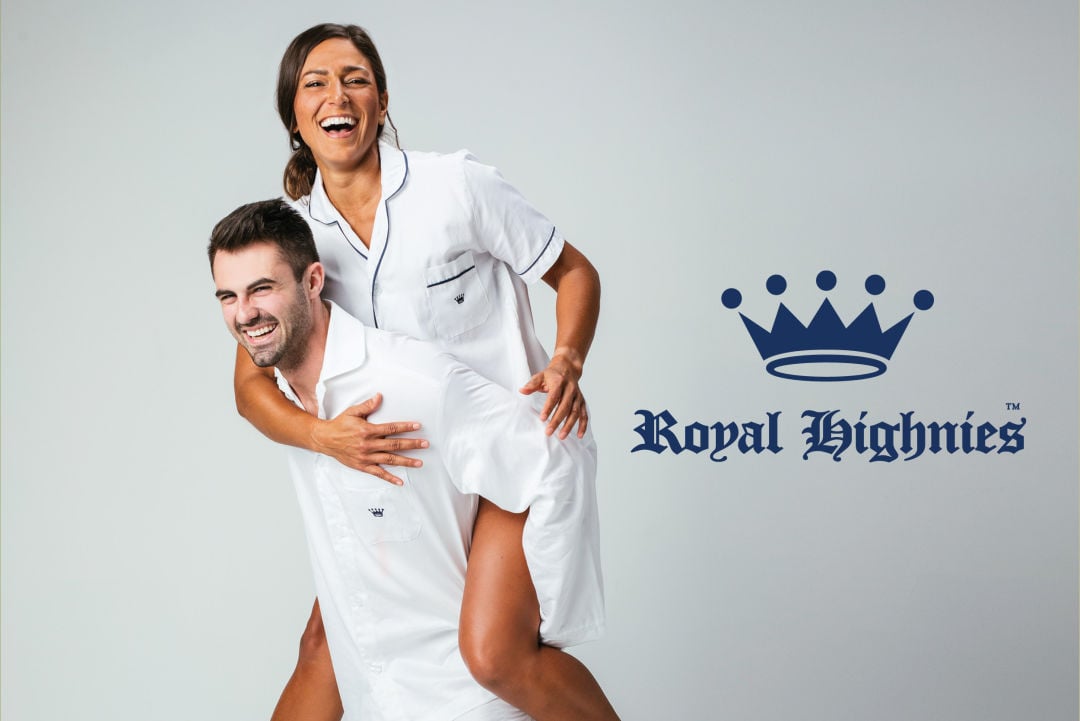The image features a light blue background with a playful yet sophisticated vibe, likely representing an advertisement for the Royal High Knees brand, which appears to specialize in loungewear or pajamas. On the right-hand side of the image, there is prominent branding that includes a blue crown logo, a halo with five dots above it, and the words "Royal High Knees" in an elegant, royal font, complete with a trademark symbol.

Centered in the composition, a man is giving a woman a piggyback ride. Both are dressed in white loungewear adorned with the same blue crown logo on their front shirt pockets, suggesting they are modeling the brand's products. They are both smiling joyfully and looking directly at the camera, exuding a sense of fun and comfort. The woman's right hand rests on the man's chest, while her left hand holds onto his arm, which supports her legs. Their relaxed and happy demeanor captures the essence of the brand, indicating that Royal High Knees loungewear is designed for both comfort and enjoyment.